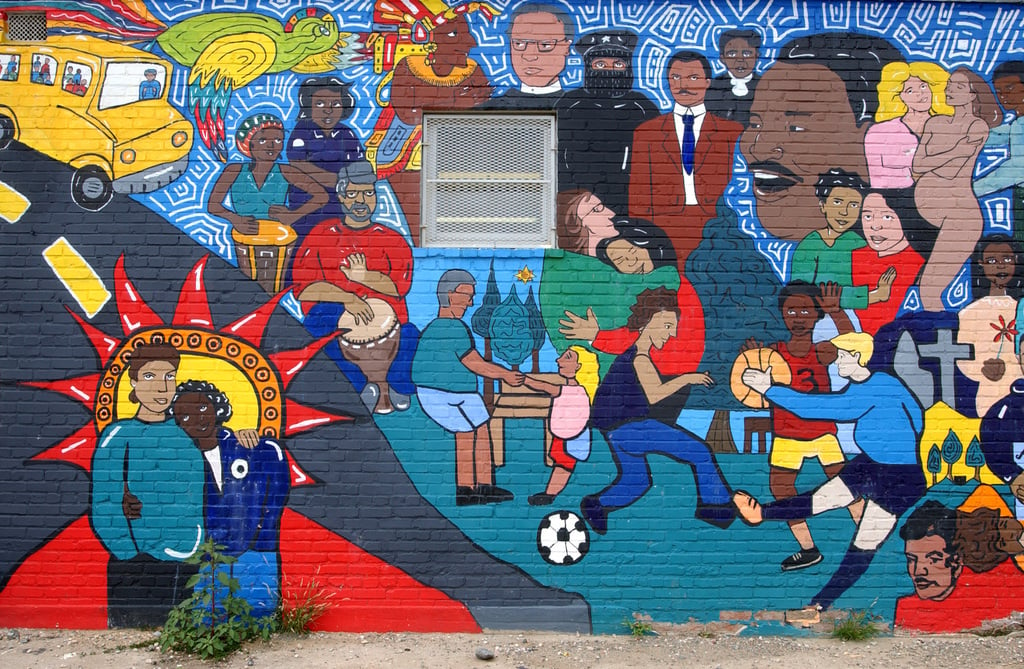This vibrant and detailed mural adorns the side of a brick building, with the image dominated by a colorful scene that spans nearly the entirety of the wall. The mural is segmented into various thematic sections, all paying homage to African-American culture and history. 

In the top left corner, a yellow school bus is prominently depicted, driving along a dark asphalt road marked with yellow lines. Below the bus, two individuals, one with brown hair in a turquoise sweater and black pants, and another, a black person with dreadlocks in a brighter blue jacket and jeans, stand embraced in front of a vivid red sun. This duo seems to represent unity and diversity.

Further to the right, the mural transitions into a diverse tableau against a blue background adorned with white, curly-Q decorations. Several figures are dynamically engaged in activities; some are playing soccer, while others play basketball or bongo drums. The top right corner of the mural features a pregnant woman, modestly covering her breasts with her arm. 

A significant historical nod is given to Martin Luther King Jr., whose profile is discernible among the numerous figures populating the mural, highlighting the narrative of civil rights and African-American legacy. The bottom right section includes a crucifix, subtly blending cultural and spiritual symbolism into the mural's overall message.

At the very bottom of the mural, minimal ground coverage is visible, showing some soil and weeds sprouting up, grounding the scene in a touch of natural imperfection.